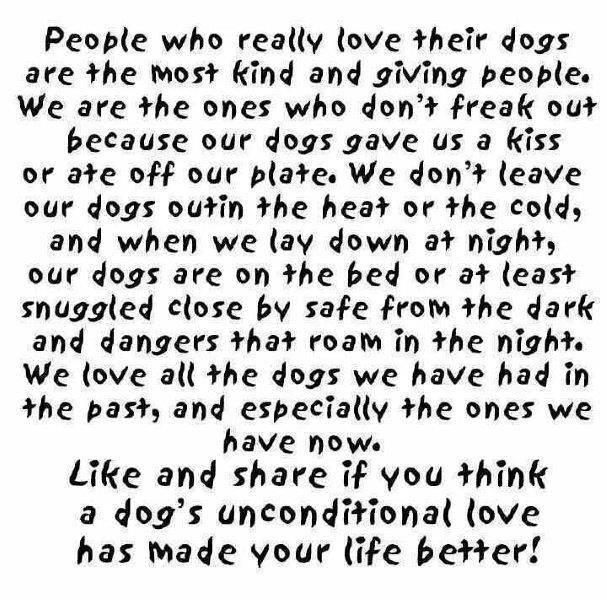The image features a heartfelt message written in a unique, almost handwritten-looking black font on a completely white background. The text reads: "People who really love their dogs are the most kind and giving people. We are the ones who don't freak out because our dogs gave us a kiss or ate off our plate. We don't leave our dogs out in the heat or the cold. And when we lay down at night, our dogs are on the bed or at least snuggle close by, safe from the dark and dangers that roam in the night. We love all the dogs we have had in the past and especially the ones we have now. Like and share if you think a dog's unconditional love has made your life better!" This simple yet evocative image, resembling an internet meme, celebrates the unconditional love between dog owners and their pets.